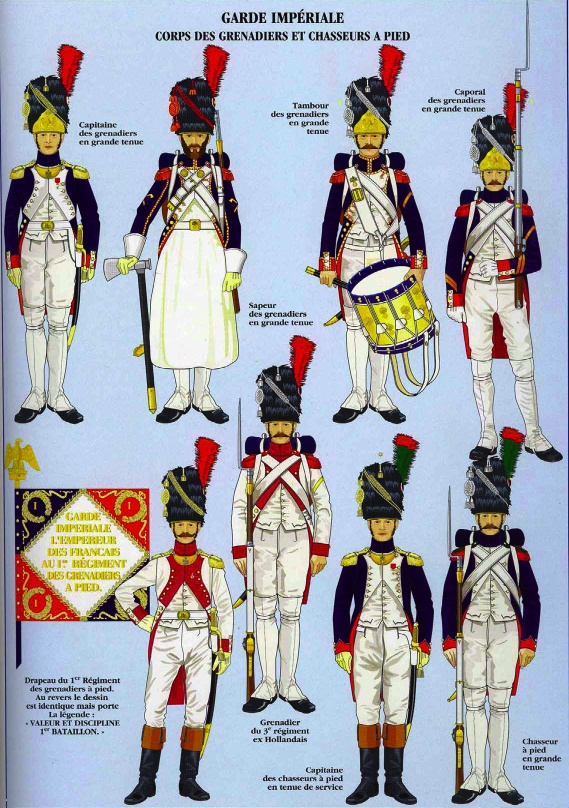The image is a detailed illustration of various French soldiers from the Garde Impériale, including the Cours des Grenadiers et Chasseurs Appelés, displayed in a stylized, almost cartoon-like manner. The top of the image features four distinct soldiers in elaborate uniforms. The first soldier, a captain, is dressed in white slacks and a white torso with black sleeves, gold shoulder pieces, and a tall black hat adorned with a red feather, carrying a saber. The second soldier is a sapeur, recognizable by his white kilt, similar arm and shoulder fashion as the captain but with black shoulder pieces, holding an axe and a rifle slung on his back. The third soldier, a drummer or tambour, mirrors the captain's uniform but carries a snare drum. The fourth figure, a corporal or caporal, wears an identical ensemble to the first soldier, with a tall black hat featuring a gold front, wielding a musket or rifle with a bayonet.

The bottom row continues with an array of soldiers and items. On the far left is a soldier carrying a drapeau du 1st Regiment, a flag with a red, white, and blue design and a golden eagle emblem. Next is a grenadier from the 3rd Regiment, dressed in red vests, white pants and sleeves, either red or gold shoulder pieces, black boots or shoes, and either long rifles with bayonets or swords. The third solider, another captain, wears a black overcoat, white vest, and the same white pants. The final figure in the bottom row is a chasseur lapide and grenadier, wearing a dark jacket, white pants, and equipped with a long rifle and backpack. The flag depicted on the bottom left features a segmented design with blue, red, and gold triangles forming a border around a central diamond shape, symbolizing the regiment’s colors and valor. The translated legend at the bottom reads: "Valor and Discipline, 1 Battalion, Grenadier of the 3rd Ex-Dutch Regiment, Captain of Foot Hunters and Service Tents, Large Foot Hunter."

The intricate details and vibrant colors emphasize the formality and distinction of each soldier's role within the Garde Impériale.